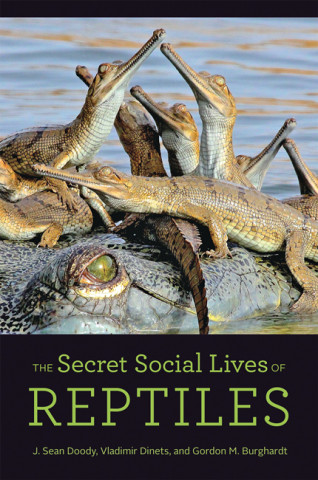This image depicts the cover of a book titled "The Secret Social Lives of Reptiles" by J. S. Doody, Vladimir Dents, and Gordon M. Berghind. The design features a square, color photograph positioned at the top of the cover with a black background above and below it. The photograph intriguing shows approximately eight tiny baby caimans or crocodiles playfully resting on the broad snout of a larger parent caiman, whose eye is prominently facing the viewer. The large reptilian snout occupies the entire width of the photograph at the bottom, emphasizing its protective and imposing presence. Below the photograph, on a black band, the book's title is vividly displayed in bright green text, followed by the authors' names. The cover's color scheme includes grays, blacks, greens, lighter browns, lime greens, and blues, contributing to an eye-catching and realistic representation that encapsulates the intriguing social behaviors of these reptiles.